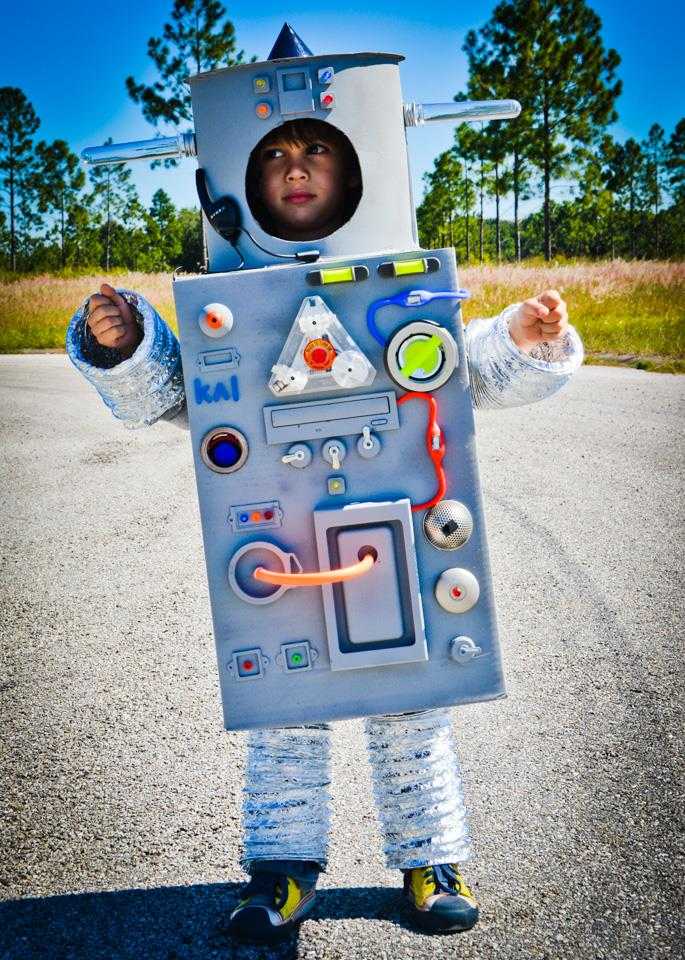This color photograph captures a young boy, estimated to be between 5 to 9 years old, dressed in an elaborate homemade robot costume. The costume is primarily constructed from cardboard boxes, papier-mâché, and insulation material, all painted in a grayish-silver hue. The head of the robot features an opening that reveals the boy's face, and is adorned with metal bars protruding from either side and a headpiece with a small microphone. The boy's arms and legs are encased in a silvery, tube-like material resembling ventilation ducts, adding to the robot effect.

The body of the robot costume is detailed with various painted controls in fluorescent green and bright orange. Notably, there are several buttons, wires, and even a flux capacitor-like device, with the name "KAI" written prominently in blue on the front. The boy is slightly leaning to his left as he stands on an asphalt driveway. The background showcases a clear blue sky and tall trees, providing a natural contrast to the metallic, playful creativity of the robot costume.